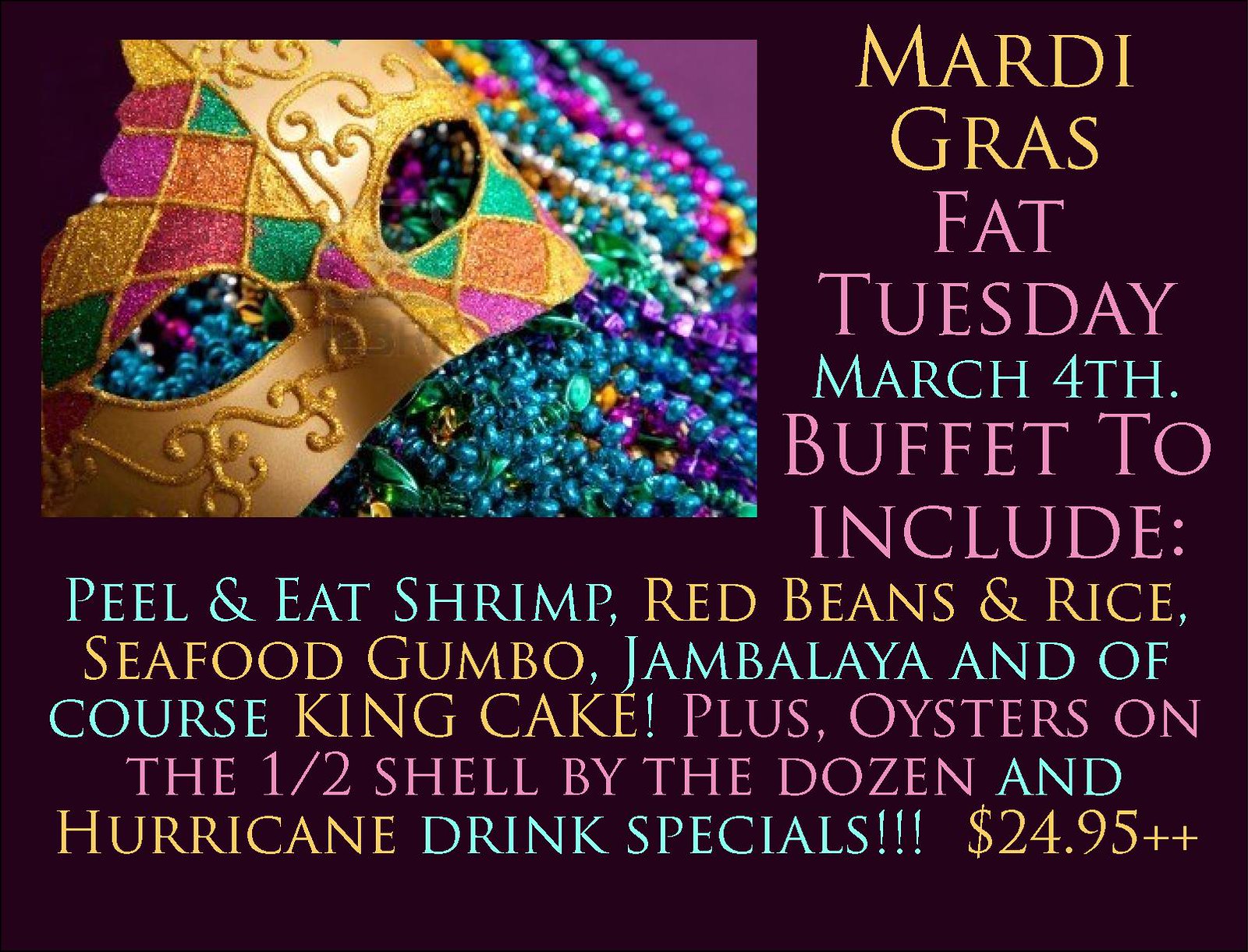This is a vibrant and detailed advertisement for a Mardi Gras celebration on Fat Tuesday, March 4th, likely promoting a restaurant's buffet. The ad features a black background with cycling multicolored text in shades of yellow, pink, and teal, displayed on the right third of the top half and encompassing the entire bottom half. On the upper left side, there is a prominent gold theater mask decorated with diamonds in maroon, fuchsia, green, orange, and yellow in the upper left and lower right quadrants. The mask is adorned with intricate gold scrollwork and rests on a pile of colorful Mardi Gras beads in hues of blue, green, purple, white, and gold. The buffet details are vividly listed in pastel colors, including peel-and-eat shrimp, red beans and rice, seafood gumbo, jambalaya, king cake, oysters on the half shell by the dozen, and hurricane drink specials, all for $24.95. The advertisement, framed in a wide vertical rectangular shape, exudes the festive and lively spirit of Mardi Gras.